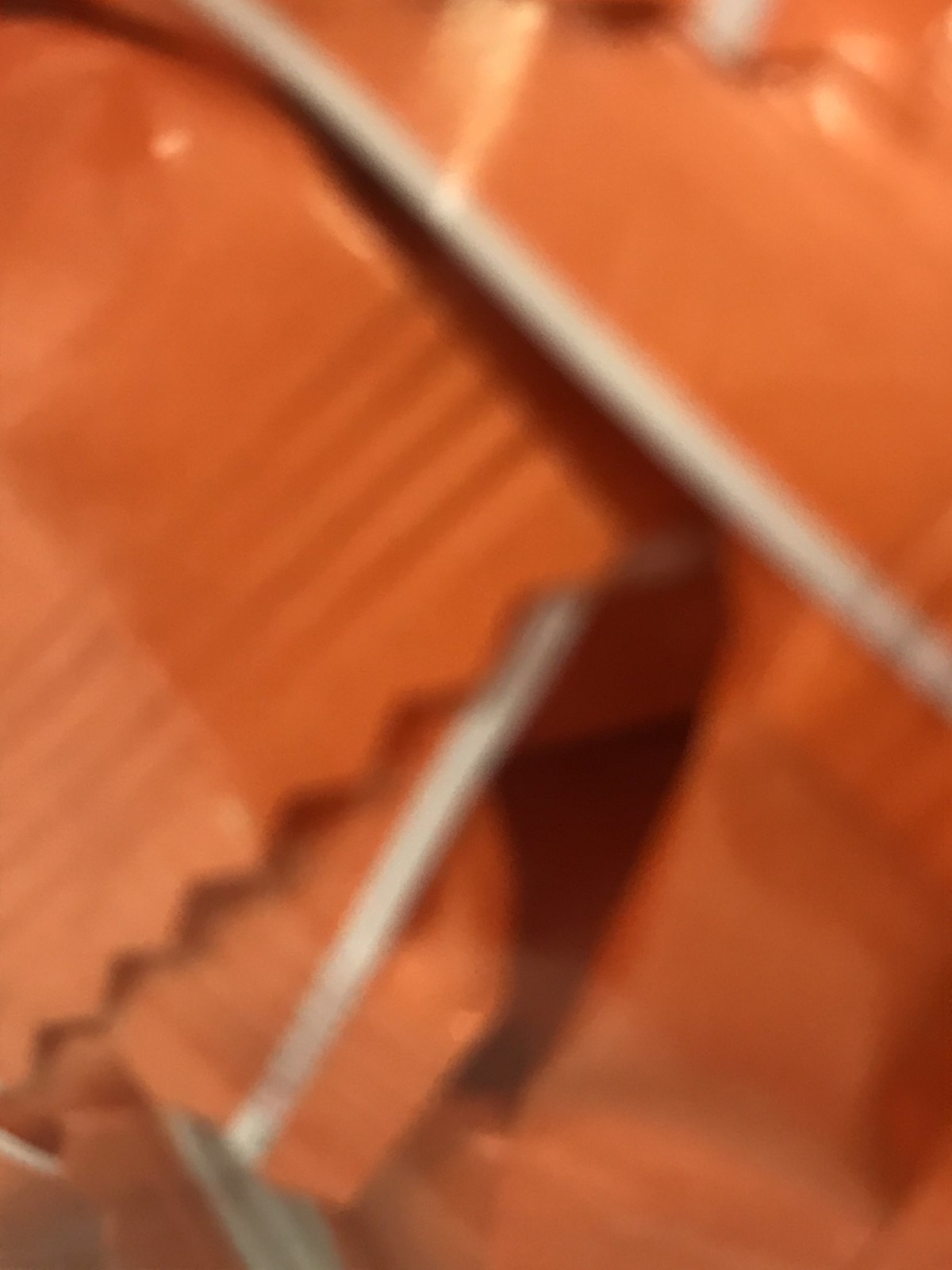This close-up photograph showcases a disorganized stack of orange and brown snack or candy bar wrappers, featuring distinctive jagged and scalloped edges. The wrappers, which may also resemble plastic chip bags, are piled haphazardly, creating a chaotic yet intricate visual. Running vertically and diagonally across the orange background, thin black lines and indented patterns add texture. Some edges of the wrappers display a white trim, further adding to the complexity. The central part of the image is notably darker, drawing the eye to the dense, shadowed middle of this slightly blurry, zoomed-in depiction.